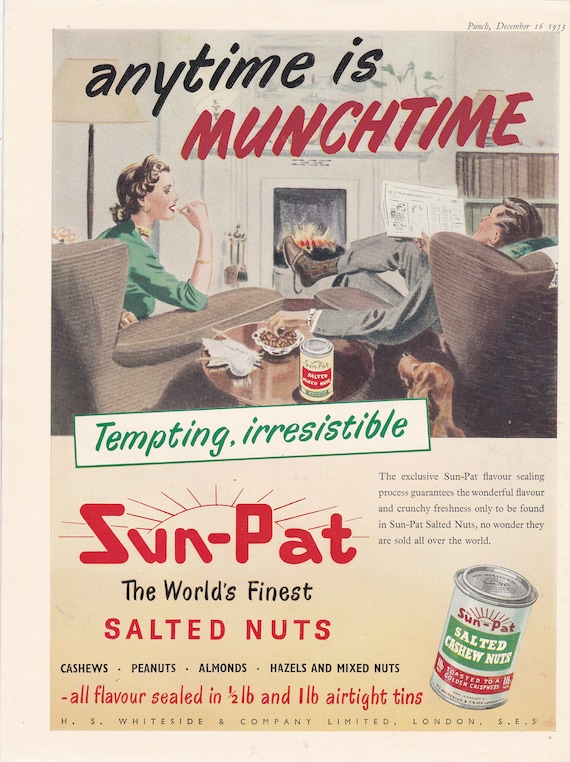This is a vintage advertisement from a magazine dated December 16th, 1953, promoting Sun-Pat salted nuts. The scene illustrates a cozy, domestic setting with a white couple sitting in front of a small fire in their living room. The couple, depicted in a colored pencil style, are seated in armchairs angled towards a brown side table. The woman, dressed in a green dress with sleeves up to her elbows, is delicately placing a nut in her mouth. Her right arm rests on the chair's armrest. The man, dressed in a gray suit with brown socks and slippers, reads a newspaper held in his right hand while reaching with his left hand into a glass bowl of nuts on the table. Next to the bowl is a can with a red label showcasing the advertised product.

A golden retriever sits behind the man's chair, adding to the homely atmosphere. The fireplace and mantel are stark white, in contrast to the vivid yellow flames.

The top of the ad displays the slogan "Anytime is munch time" in black and red text. Below the illustration, within a white textbox, it reads "Tempting, irresistible" in green, followed by "Sun-Pat" in thick, bold red letters. Further text in black and red promotes the world's finest salted nuts, listing varieties such as cashews, peanuts, almonds, hazelnuts, and mixed nuts, all sealed in half-pound and one-pound airtight tins.

An illustrated can of Sun-Pat salted cashew nuts is shown prominently, featuring a white base with a green label and red text, including the brand name "Sun-Pat" with a sunbeam design. The bottom of the can reads "Toasted to a golden crispiness." The metal sheen of the can’s lid completes the classic look of this mid-century advertisement.